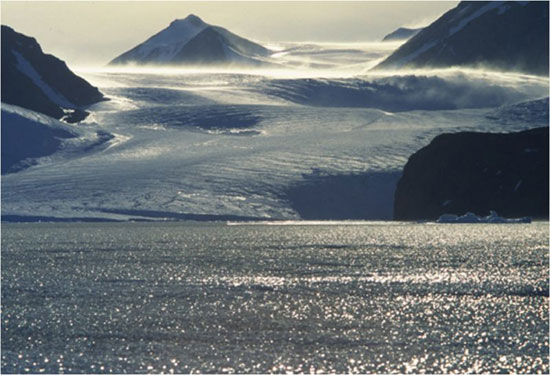The image captures a breathtaking icy landscape where the lower half glistens with either ice-covered water or icy land. This reflective surface mirrors the bright sunlight, creating a dazzling effect. Moving upwards, the scene transitions into snow-covered hills, amidst which black rocks peek through, hinting at the rugged terrain beneath. The middle and top sections of the image showcase several imposing mountains with peaks emerging from colossal snow banks, shrouded partly by a misty fog. The photo, taken during daylight, features a palette dominated by whites, grays, and light blues. The sun's rays illuminate the scene, adding a silver shimmer to the snow and creating a stark, almost desolate beauty. The mountains are predominantly white with sporadic dark patches where the snow has not settled, enhancing the dramatic contrasts within the image.